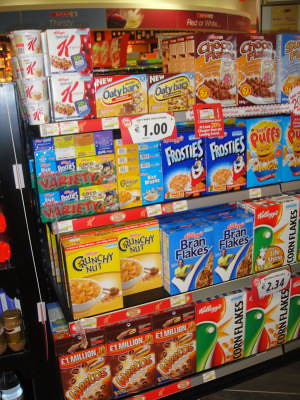This is an image of a grocery store shelf display featuring a variety of breakfast items. The display consists of a metal cart with four shelves, ranging from close to the ground to the top shelf. The cart primarily holds an assortment of cereals, including both name brands like Kellogg's Corn Flakes, Bran Flakes, Crunchy Nut, Frosties, Special K, and Count Chocula, as well as off-brands. The cereals come in various sizes, from small individual boxes to large family-sized packages, and are packaged in colorful boxes of yellow, red, blue, beige, and brown. In addition to the cereals, there are also cereal bars, such as nut and oat bars, placed on the top shelf. The display cart is adjacent to another shelf, which appears to hold jars of gravy. The prices on the items seem to be marked in euros, with some discounts noted. The setting appears to be a somewhat eclectic grocery store.